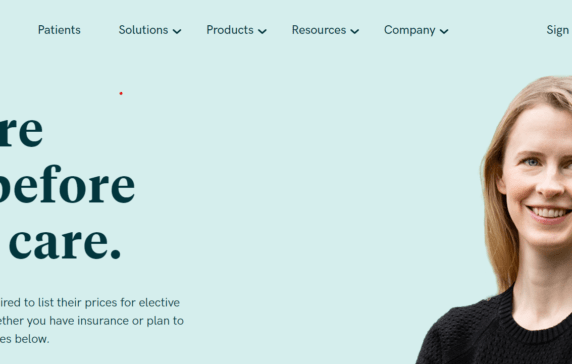This image captures the top portion of a website with a light greenish-grayish-blue background. Prominently displayed at the top are several tabs labeled "Patients," "Solutions," "Products," "Resources," and "Company," each featuring drop-down icons for additional options. In the top right corner, there is a "Sign In" option for account access. Towards the bottom left, partially visible black text appears in bold, followed by regular black text underneath. The right side of the image showcases a woman with light brown hair, wearing a black sweater. She is smiling warmly, adding a personable touch to the website's design.